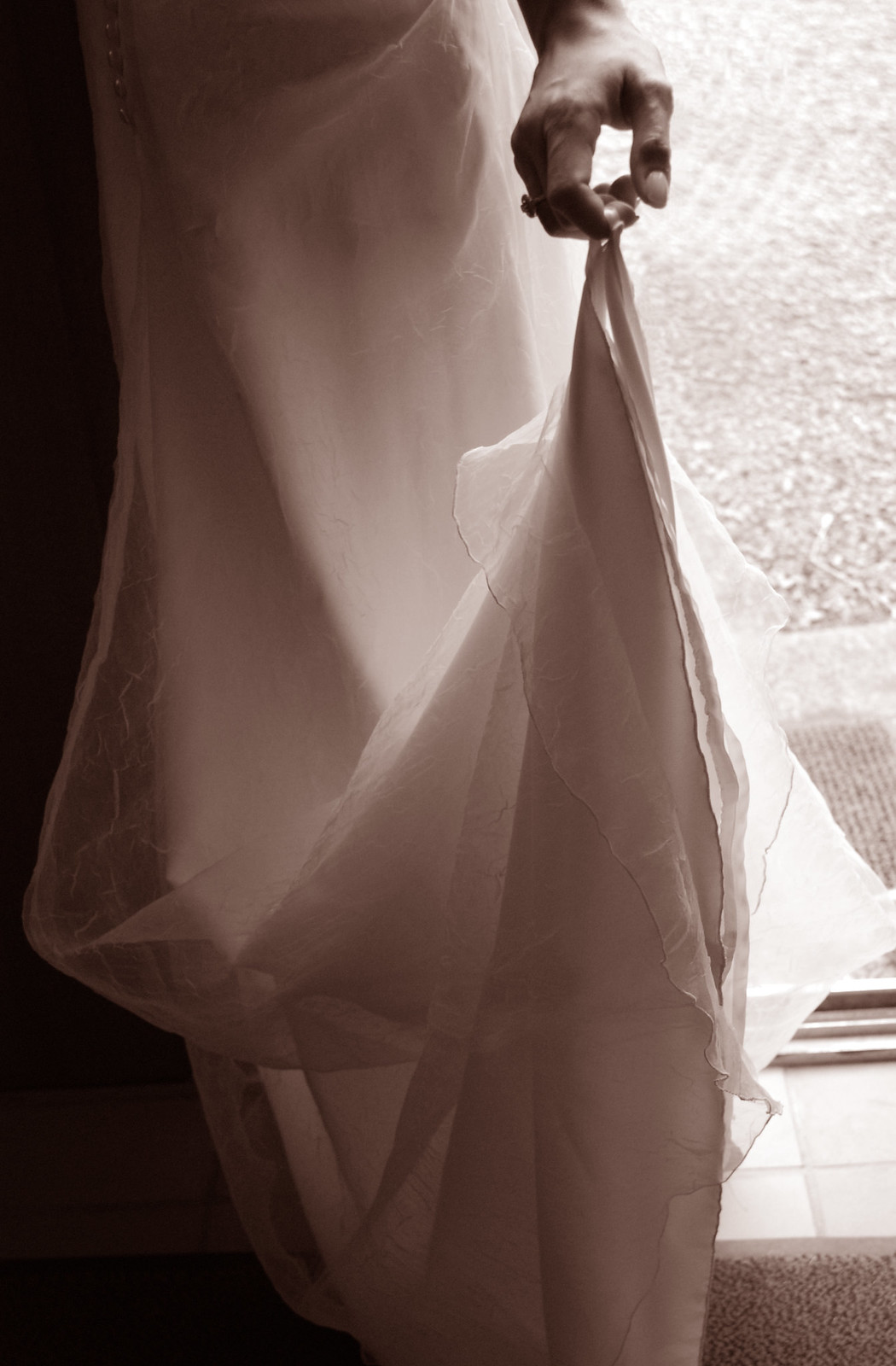The photograph is a close-up, black-and-white image capturing the lower third of a woman, identified primarily by her hand holding up the corner of her dress. The dress, which appears to be a light color rendered dark by the monochrome lighting, forms a triangular shape as it is lifted. The setting includes a carpeted floor with visible tiles behind, suggesting an indoor environment, potentially in front of a sidewalk or window for optimal lighting. The scene includes a variety of textures and colors, such as tan, gray, and silver, enhancing the visual depth. The image, centered around the fabric of the dress, is devoid of any text and seems to portray a serene, indoor moment, possibly during the day.